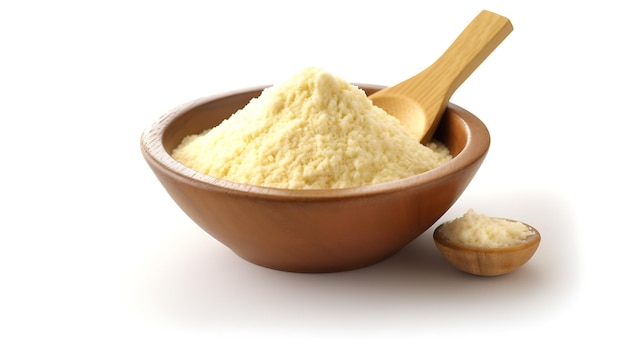This image is a detailed, color photograph in landscape orientation featuring two wooden bowls set against a completely white background. The larger bowl, located to the left, has a darker brown hue and contains a wooden spoon of a lighter wood tone. The spoon is angled with its handle pointing toward the top right corner of the image. Inside this bowl is a mound of a slightly off-white, lumpy powder, which is piled up into a small peak. This powder looks similar to unmixed instant mashed potatoes or a flour-like substance. To the right of the larger bowl, and very close to it with just a slight space in between, is a smaller bowl of a slightly lighter wooden color, mimicking the coloration of the spoon. This smaller bowl also contains the same off-white powder, which almost overflows but does not form a distinct shape. Both bowls have a wider top and taper towards the bottom, and they cast a subtle gray shadow on the flat white background, adding depth to the image. The overall style is realistic and focuses on food photography with a representational approach.